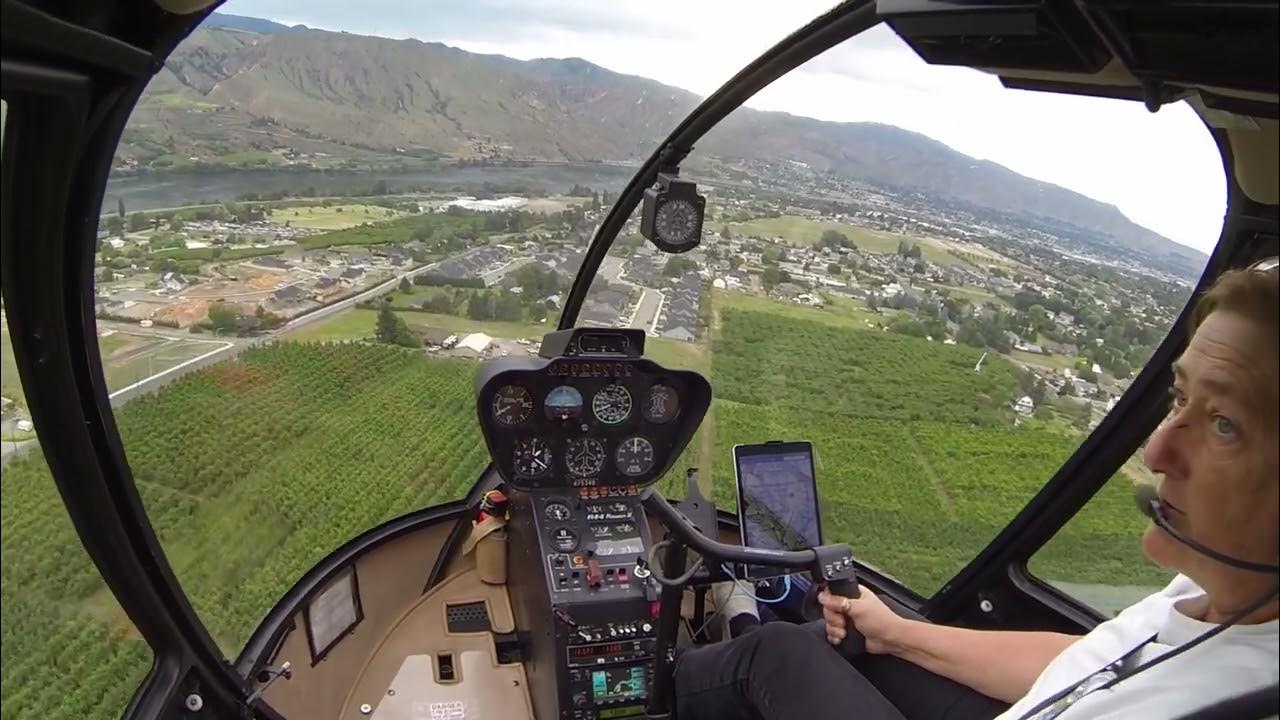In this detailed photograph taken inside a small helicopter, we see an airline pilot located in the lower right-hand corner of the frame. He is wearing a white shirt, black pants, white shoes, and a headset with a microphone positioned at his mouth. His right hand is firmly placed on a black, curved steering column that connects to a central control panel. This intricate dashboard is populated with numerous dials and switches organized into sections; at the top, there are four main dials, followed by three dials below, and beneath those lies a box-shaped or trapezoid-shaped array of additional controls. Adjacent to the main panel, on his right, is a large tablet displaying a detailed map for navigation purposes. 

Ahead of the pilot, through the expansive clear glass windows, the exterior landscape unfolds. The helicopter hovers above a patchwork of lush green fields and farmlands interspersed with square plots. Further in the distance, a sprawling town or city is visible, framed by majestic mountain ranges beneath a blue sky dotted with white clouds. The pilot himself is gazing intently off into the horizon, focused on something beyond the frame, giving a sense of calm and control on what appears to be a fairly clear and picturesque day for flying.